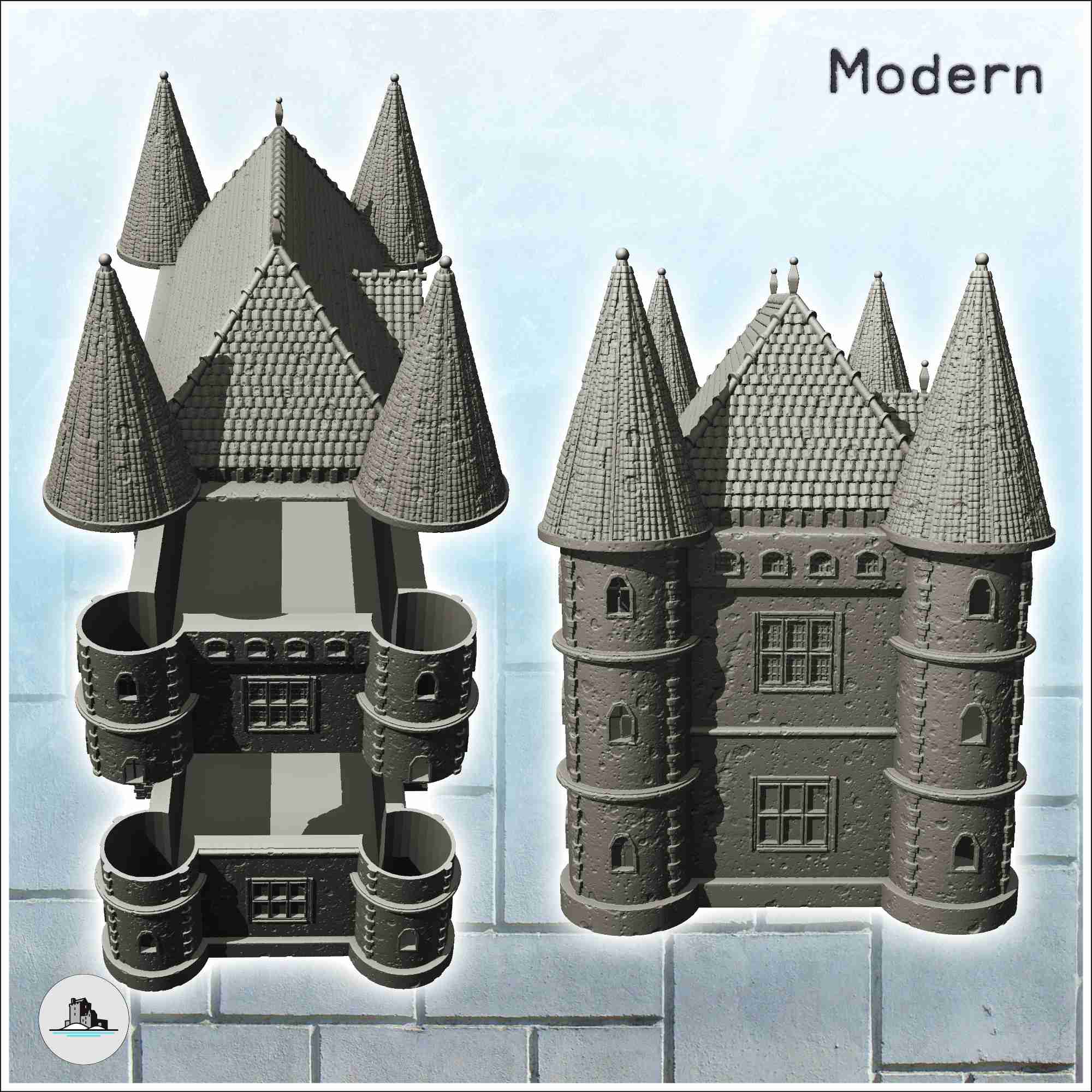The image showcases two detailed 3D renderings of a Victorian-style house design with cylindrical columns, likely containing spiral staircases. The house, predominantly in shades of gray with a conical roof, stands prominently in the middle right of the image. Adjacent to it, on the left, is a deconstructed version of the same house, segmented into three levels: the roof, the second floor, and the base, illustrating the architectural layers. The backdrop transitions from a blue sky at the top to a stone brick pattern in white and gray towards the bottom. The word "Modern" appears in black text at the top right corner, while a logo is positioned at the bottom left corner. The overall setting seems to serve as an architectural showcase, emphasizing the modern yet Victorian-inspired design.